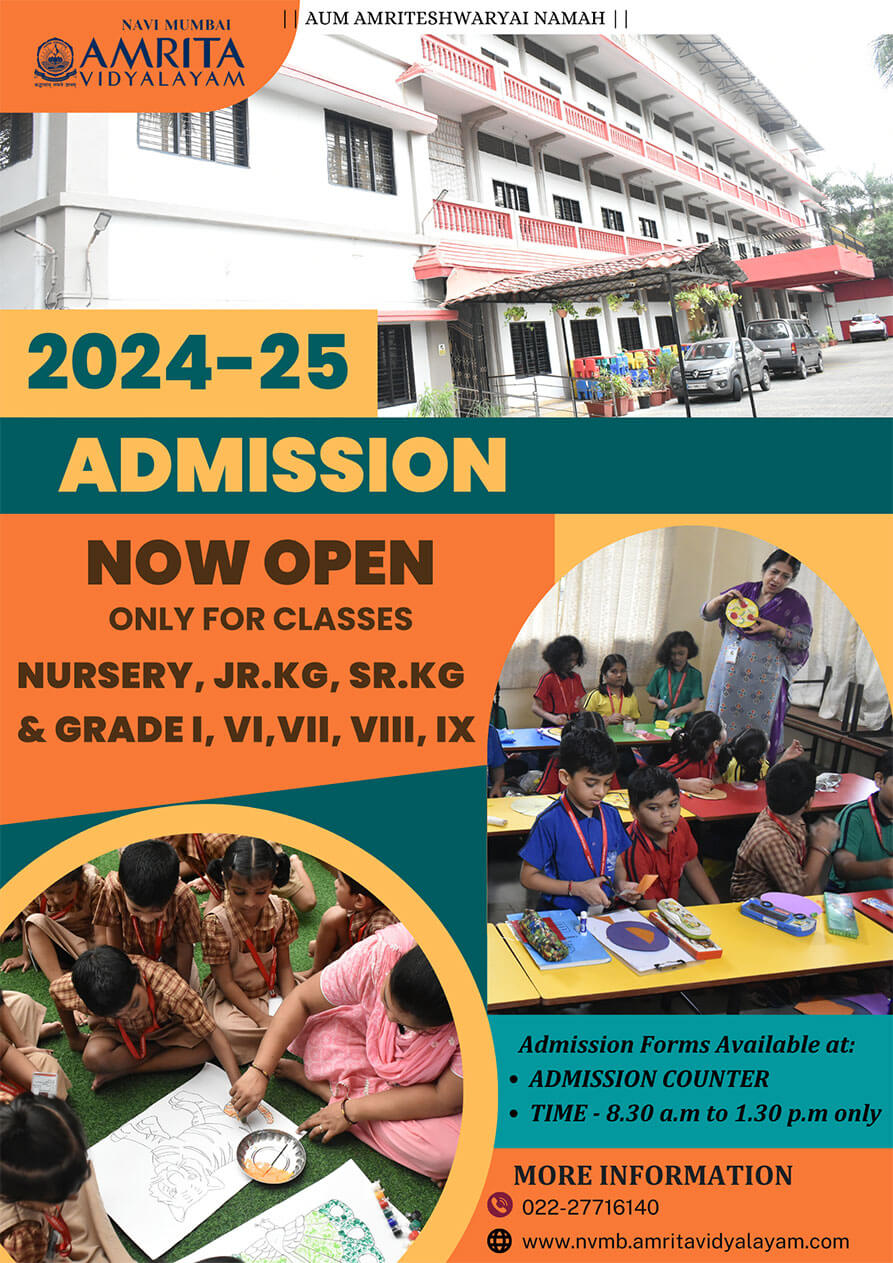**Amrita Vidyalayam Mumbai Preschool and Nursery School Admissions Flyer**

At the top corner of the flyer, the institution’s name, Amrita Vidyalayam, is prominently displayed. Below the name, the text "24-25 Admissions" is visible, indicating the upcoming academic year's enrollment. The upper third of the flyer features a hero image of the school, which bears a resemblance to an American motel.

The bottom two-thirds of the flyer contain important admission information. The middle section announces that enrolment is now open for Nursery, JRKG, SRKG (Junior and Senior Kindergarten), and Grades 1, 4, 6, 7, and 9. This section also includes two heartwarming images of children engaged in creative activities with a teacher; in one image, the children are drawing, while the other image shows them coloring a tiger.

In the lower right corner, the flyer gives additional details: Admission forms are available at the admissions counter from 8:30 a.m. to 1:30 p.m. only. For more information, interested parties are encouraged to call 022-277-16140 or visit the provided website.